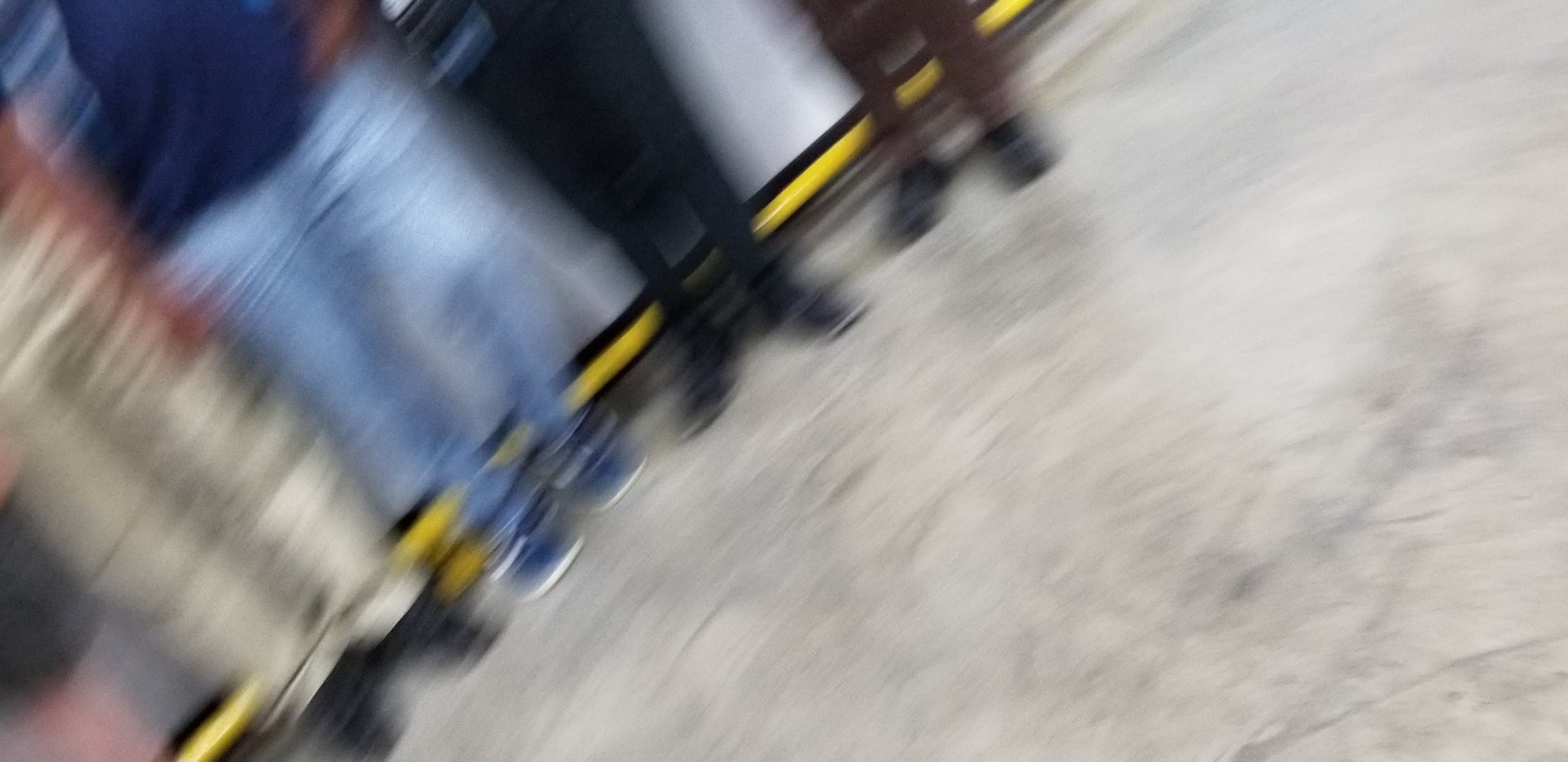This image shows the lower halves of four individuals standing closely together on a dirty, scratched-up gray floor with darker gray marbling. The angle of the photo makes them appear to be standing diagonally, though they are actually facing straight ahead. The shot captures the first two people from the waist down, the third from the waist down, and the fourth from the calves down. To the right, behind them, a thin yellow line outlined in black marks the floor, adding a cautionary element, possibly indicating they are waiting for a bus or train. The floor is notably dirty, with black scratches and lines. The first person on the left wears white pants and black shoes, the second person sports a blue shirt with blue jeans and blue shoes, the third individual has black pants and black shoes, and the fourth person is clad in dark brown pants and black shoes. The blurred image adds a sense of mystery, making finer details hard to discern and hinting at a school or public setting due to the blue wall above the yellow and black border.